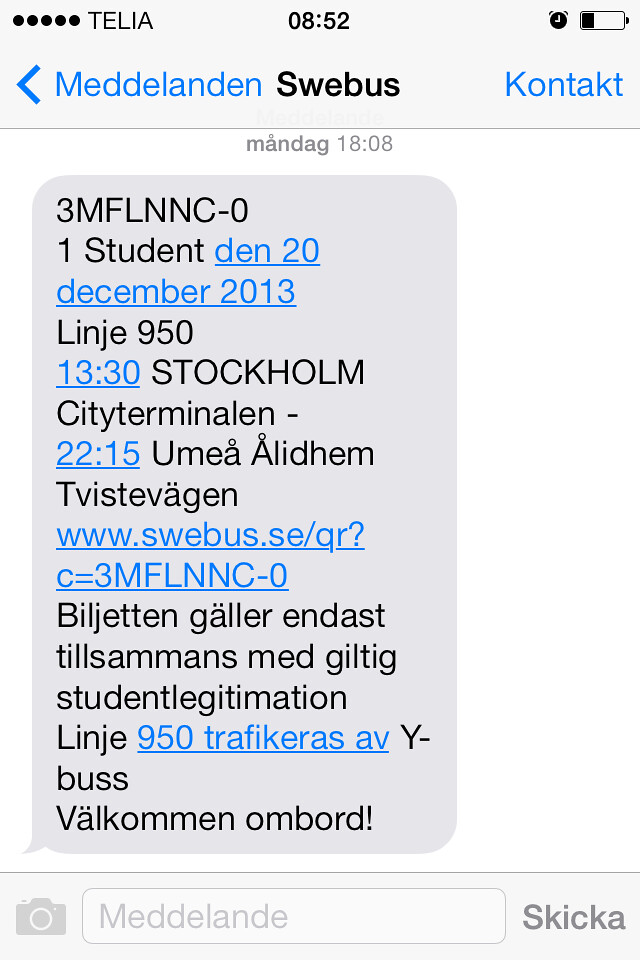The image is a screenshot of a text message conversation on a smartphone, primarily in Swedish, and taken at 8:52 AM. At the very top, the phone displays standard indicators such as the service provider "Telia," battery life showing about one-third charge, and an alarm clock icon indicating an alarm is set. The header also includes service-specific info with "Swebus" in black font, suggesting the text might be related to bus or transport services in Sweden, particularly mentioning "Stockholm." The message appears to discuss details about traveling to Stockholm, evident from the use of the capitalized "Stockholm" within the message, along with a website link to Swebus, and dates including December 2013, and multiple time stamps. At the bottom of the screen, there are standard messaging app features including an input field for new messages, a send button, and an attachment icon.